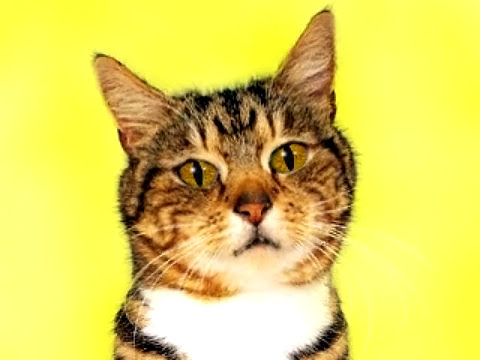In the image, set against a bright yellow background with a faint white hue, a tabby cat is prominently featured from the neck up, centered perfectly in the frame. The cat's fur showcases a mix of black stripes and various shades of brown, with a distinctive white chest. Black stripes are noticeable running down the middle of its head and to the sides near its eyes, which are strikingly green with black pupils. The cat's ears, which are pointed and brown, sit alert atop its head. It has long, white whiskers that sprout from small black spots on its snout. The cat's nose is pink, adding to its expressive face, which is caught in a moment that makes it look slightly confused or upset, perhaps due to the timing of the photograph. The background is a solid yellow, creating a striking contrast that draws attention to the cat's intricate fur patterns and vivid eyes.